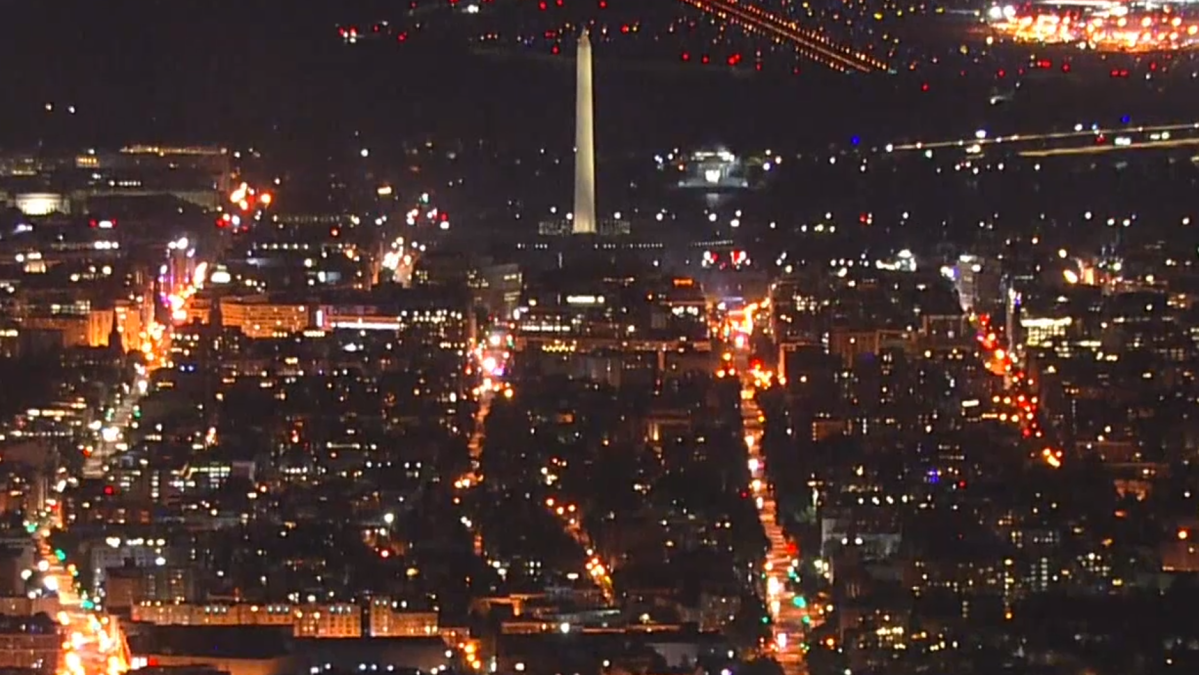This nighttime aerial photograph, likely taken from a helicopter, captures the Washington Monument in Washington, D.C., prominently positioned in the top center of the image. The monument is brightly illuminated, standing tall amidst the surrounding darkness. The cityscape below is a grid of largely dark buildings, punctuated by streetlights and the headlights of cars, which create a warm orange-red hue across the roads. These headlights carve glowing paths through the city, highlighting the structured division of buildings by the streets. In the distance, closer to the horizon, faint lights hint at an airfield or airport, adding another layer of depth to this nighttime urban scene.